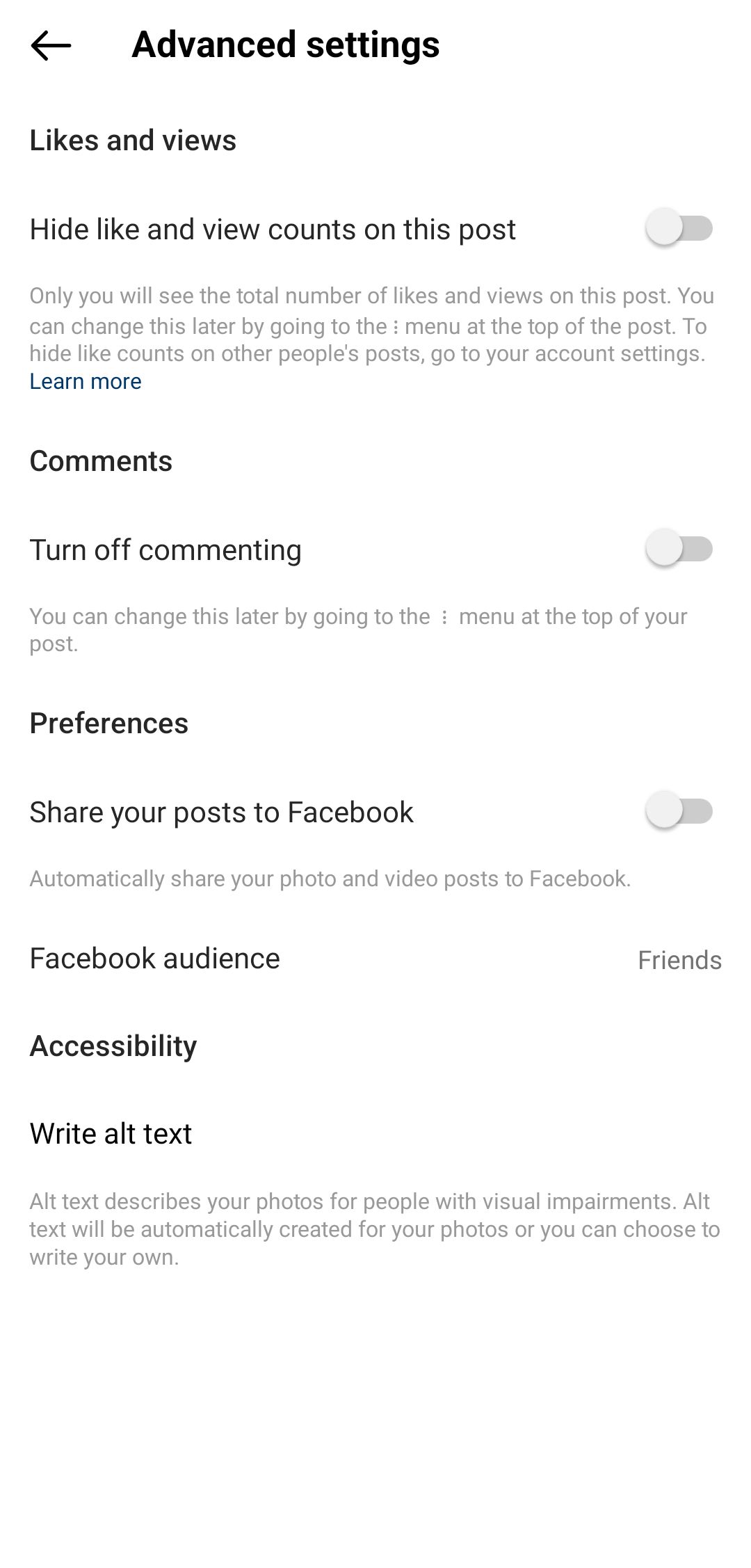This image is a screenshot of an advanced settings screen on a device. At the top of the screen, "Advanced Settings" is displayed, along with a left-pointing arrow that allows users to navigate back to the previous page.

The menu items listed consecutively down the screen include:

1. **Likes and Views:**
   - *Hide like and view counts on this post*: A toggle button allows users to turn this setting on or off. When enabled, only the user will see the total number of likes and views on their post. This setting can be adjusted later through the options (three dots) menu at the top of the post.
   - *Additional Information*: To hide like counts on other people's posts, users are directed to go to their account settings. A "Learn More" link provides further details.

2. **Comments:**
   - *Turn off commenting*: Another toggle button allows the user to disable comments on their post. This can also be changed later via the options menu at the top of the post.

3. **Preferences:**
   - *Share your posts to Facebook*: A toggle button to enable or disable the automatic sharing of the user's photo and video posts to Facebook.
   - *Facebook Audience*: Set to "Friends," this indicates the default audience for shared posts on Facebook.

4. **Accessibility:**
   - *Write alt text*: Provides an option for users to describe their photos for individuals with visual impairments. Alt text can be automatically generated or manually written by the user to ensure accessibility.

The detailed, structured layout of options allows users to customize their post visibility and accessibility settings easily.